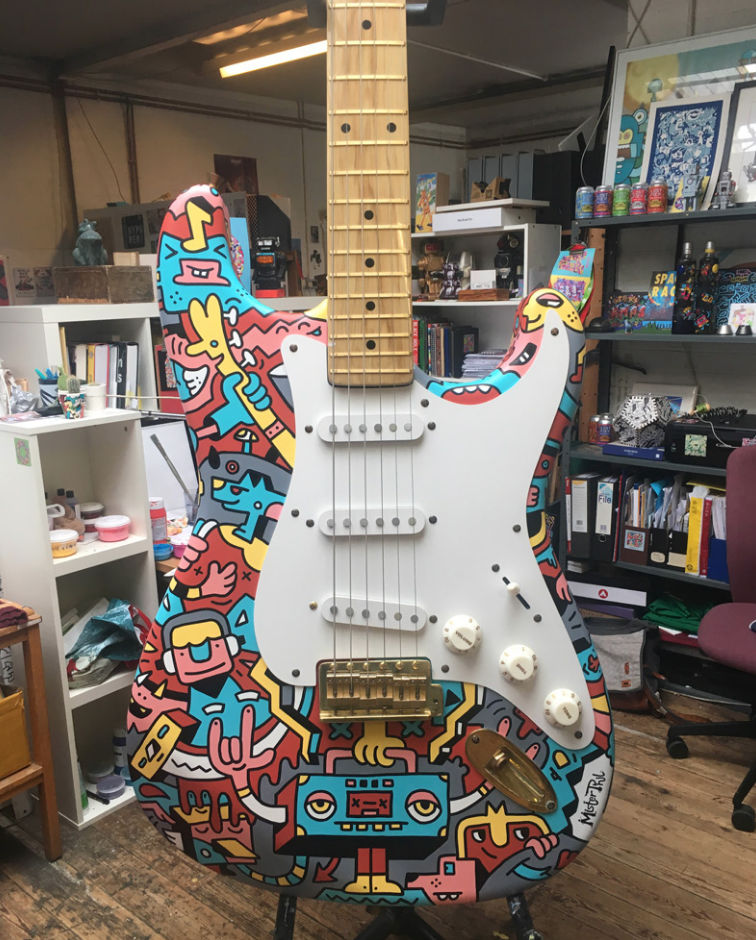The image features an electric guitar positioned upright on a stand. The top of the guitar is cut off, but at least half of the wooden neck with gold-colored frets is visible. The body of the guitar showcases a white pickguard, while the rest is adorned with vibrant, multicolored cartoonish designs. These include turquoise, pink, white, red, and blue hues, depicting an array of characters such as people, dogs, and an anthropomorphic radio with arms. One of the radio's hands is giving a peace sign, while the other is obscured behind a gold section where the strings attach. The guitar rests on a wooden floor with black stains and is flanked by a white bookshelf on the left and a black bookshelf on the right, both filled with books and various containers. To the far right, part of a swivel chair with a maroon cushion is visible. The background appears to be a workshop or hobby space, cluttered with items such as jars of paint, spray cans, drink cans, paintings, drawings, binders, papers, and figurines.